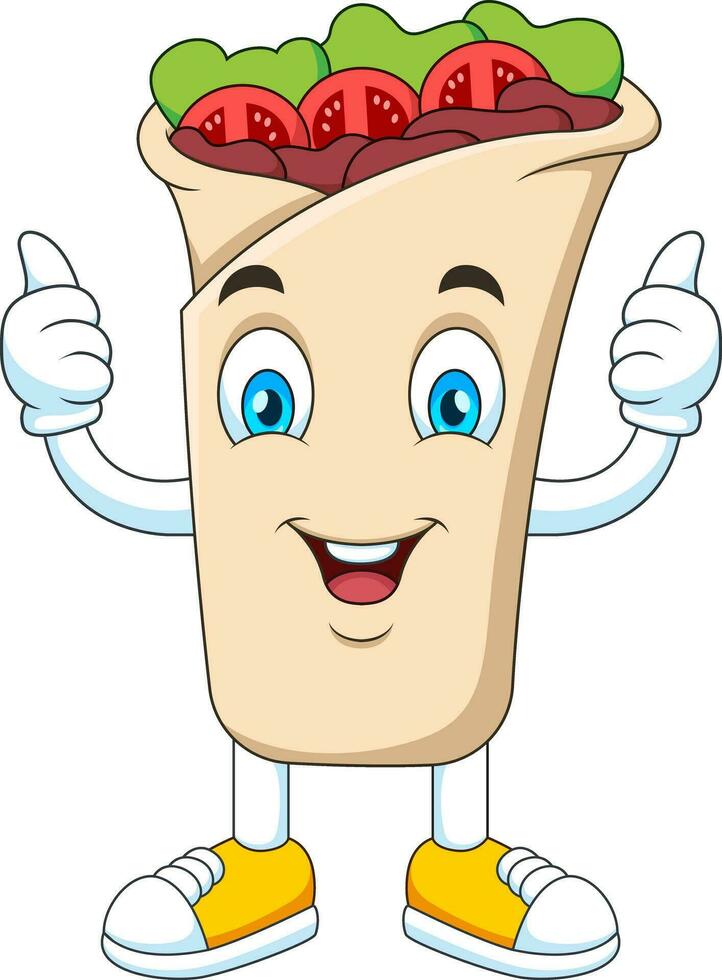This whimsical cartoon depicts a lively Fajita wrap character with a tan body made from a folded tortilla. Sporting a big, open smile, the wrap's jovial face features bright round eyes with blue centers, black pupils, and raised black eyebrows, giving it a cheerful expression. The mouth showcases a set of top teeth and a visible tongue, accentuated by curved lines at the corners that radiate happiness. From the top of the wrap, hints of its delicious inner contents—brownish meat (perhaps bacon or chicken), vibrant red tomato slices, and fresh green lettuce leaves—peek out.

The Fajita man is equipped with arms made of white PVC-like pipes ending in white-gloved hands, both posed with thumbs up, enhancing its playful demeanor. Its legs, similarly pipe-like and white, extend into eye-catching yellow sneakers with white toes, soles, and laces. The character stands against a plain white background, allowing the details of its design to pop vividly, and it bears a slight lip drawn beneath its mouth, adding to its animated charm.